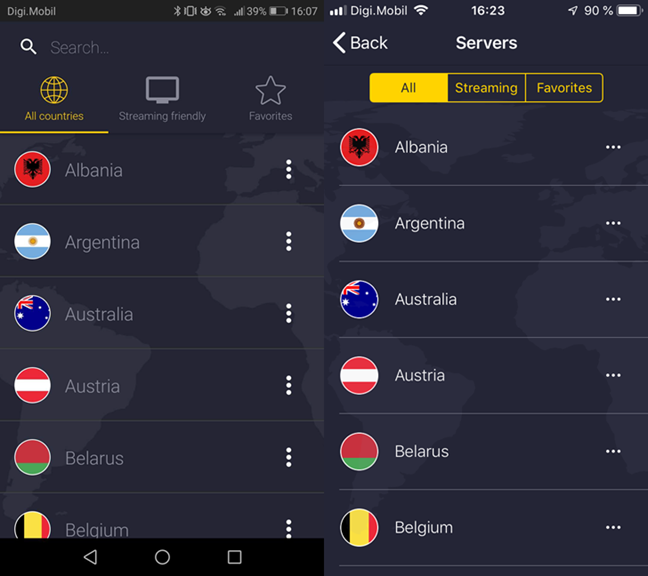This image depicts two mobile phone screens side by side, each displaying different features of a mobile application interface.

**Left Screen:**
- The top section features an empty search bar.
- Below the search bar, there are three buttons laid out horizontally:
  1. The first button displays a globe icon and reads "All Countries." It is highlighted in yellow, indicating it is currently selected. A yellow line appears beneath this button.
  2. The second button shows a TV screen icon labeled "Streaming-Friendly."
  3. The third button has a star icon with the label "Favorites."
- The main display area beneath these buttons is currently empty.

**Right Screen:**
- The top left corner features a back button.
- The central area displays the word "Servers" prominently.
- Beneath "Servers," three sections are highlighted:
  1. "All"
  2. "Streaming"
  3. "Favorites"
- Each section lists countries, represented by their flags in circular icons. The countries displayed in sequence are Albania, Argentina, Australia, Austria, Belarus, and Belgium. Next to each country's flag is a set of three dots, indicating additional options.
- The background is a silhouetted map of the globe, showcasing parts of South America, Africa, and Europe.

The overall design provides a sleek and user-friendly interface, allowing easy navigation between different server options and preferences.